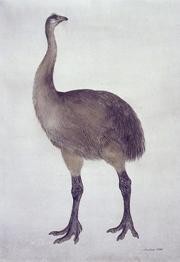The image depicts a very tall, substantial bird resembling an ostrich, characterized by its exceptionally long neck and small head. The bird's body is hefty and oval-shaped, covered in feathers, with notable distinctions in shading: its neck is light gray while its back side is a darker gray. The legs are sizable, looking almost as though they are covered in rubber or boots, and end in three dark gray talons on each foot. The muscular legs are partially feathered white near the top, transitioning to a darker, rubbery texture at the bottom. The background appears light gray, resembling watercolor paint, adding a subtle artistic touch to the photograph. Overall, the vertical, rectangular image, though small in size, conveys the bird's exaggerated proportions and distinctive features in a striking black and white palette.